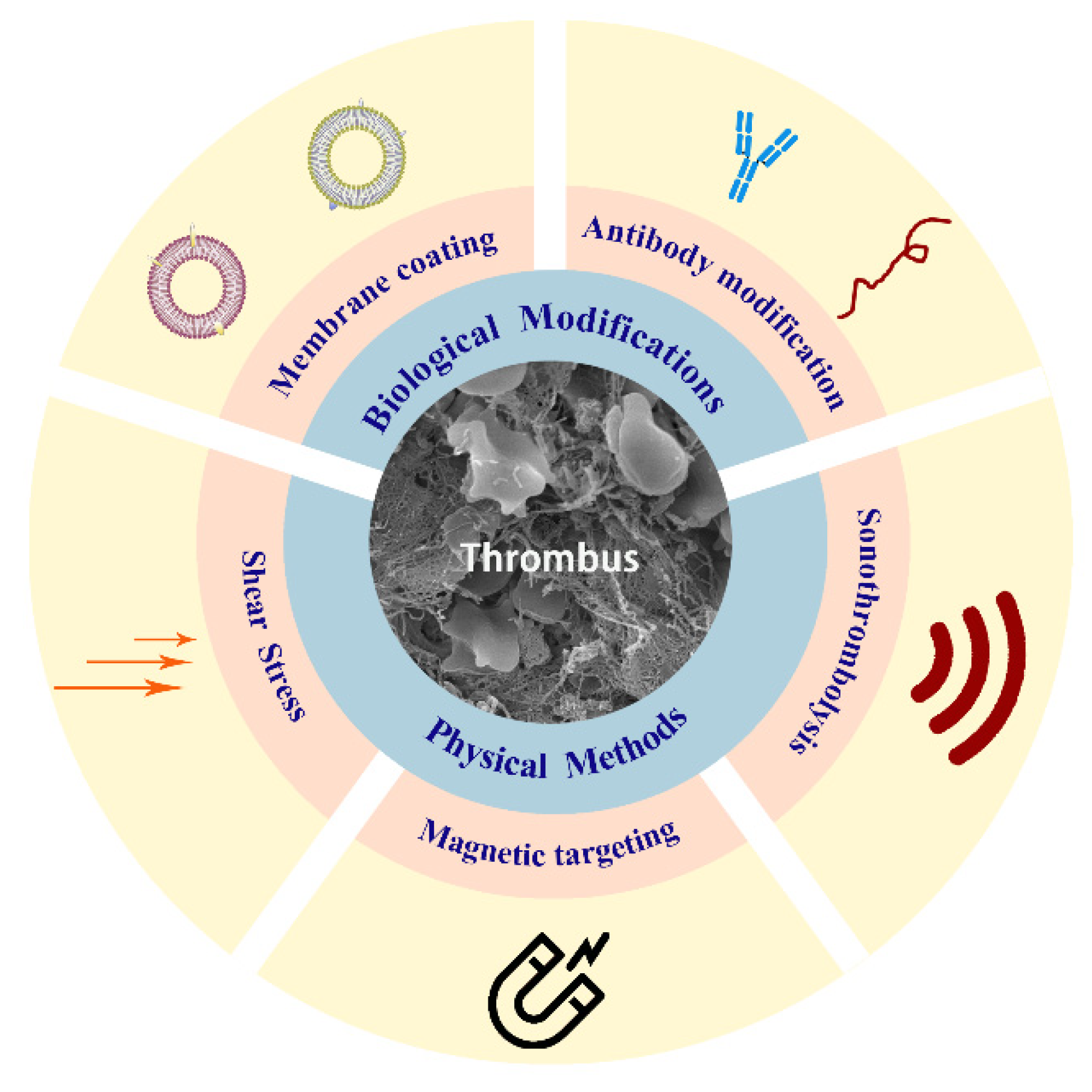The image is a detailed scientific chart with a circular design depicting various methods related to thrombus treatment. At the center, a black-and-white photograph of a thrombus (a type of blood clot) is enclosed in a yellow circular band. Surrounding this is a wider blue band labeled with the terms "biological modifications" at the top and "physical methods" at the bottom. Next, an orange circular band features key terms such as "membrane coating," "antibody modification," "sonothrombolysis," "magnetic targeting," and "shear stress." Each section is color-coded and includes relevant imagery and indicators: for example, antibodies in blue bodies and red squiggles in the yellow wedge, a magnet in the section for magnetic targeting, and red/orange arrows for shear stress. This layered, concentric circle design visually categorizes and details various thrombus intervention techniques.